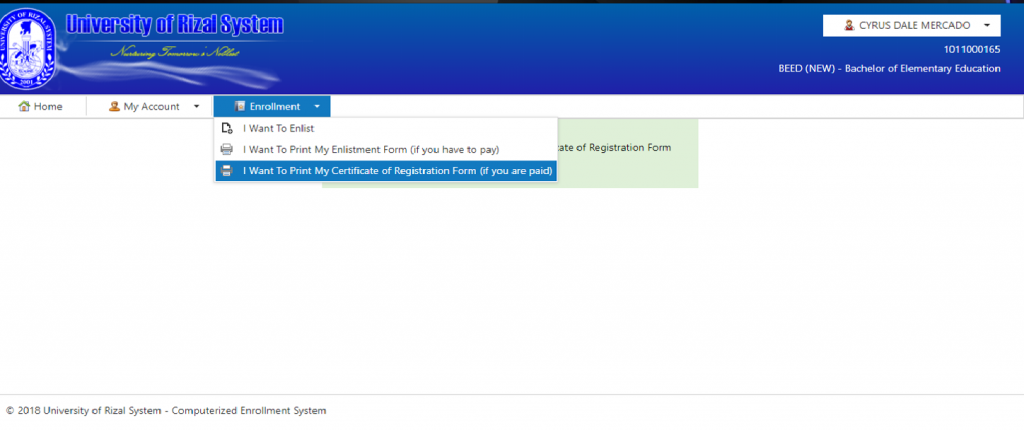This is a detailed screenshot of the University of Arizona System's website, highlighting the top section. Dominating the header is a blue banner that spans the entire width of the page. On the left side of the banner, the "University of Arizona System" text stands out in a blue font, accentuated by a subtle white glow. Adjacent to this text is the university's logo, a rounded emblem featuring a white center encircled by blue edges.

Towards the upper right corner of the banner, there is a search bar labeled "Cyrus Dale Mercado" accompanied by a drop-down arrow, indicating additional options or a user menu. Directly beneath this, a numerical identifier "101000165" is displayed, likely representing a student ID or reference number. Further below, the text "BEED (new)" is visible, denoting the Bachelor of Elementary Education program.